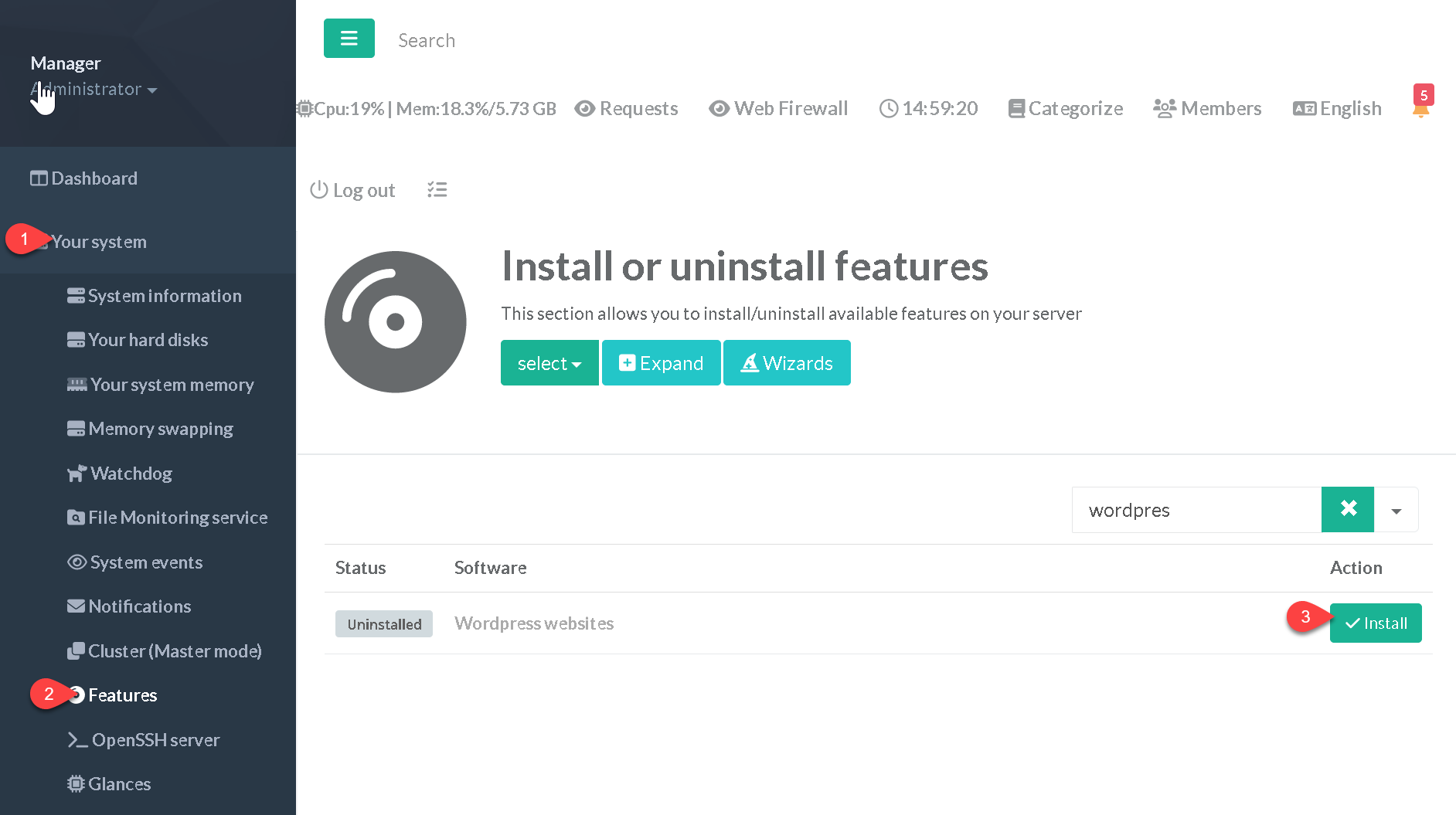The image showcases a computer program interface with a predominantly white background. On the left side, there's a prominent vertical navigation bar featuring various options. At the top of this bar, the word "Manager" is displayed in white text, followed by "Administrator" with a drop-down arrow beside it. A cursor, shaped like a hand with a pointing finger, hovers over the word "Administrator."

Below "Administrator," the navigation bar lists "Dashboard" and "Your System," accompanied by a red marker with a white number "1" inside. The following sections include "System Information," "Hard Disks," "Memory," and "Notifications."

A bold section labeled "Features" also has a red marker with a white number "2" next to it. The rest of the interface is mostly white, dominated by the main content area which displays the heading "Install or Uninstall Features." Alongside this heading is a grey disk icon with white details. Several buttons are available for user interaction, offering options to expand, select, or uninstall features.